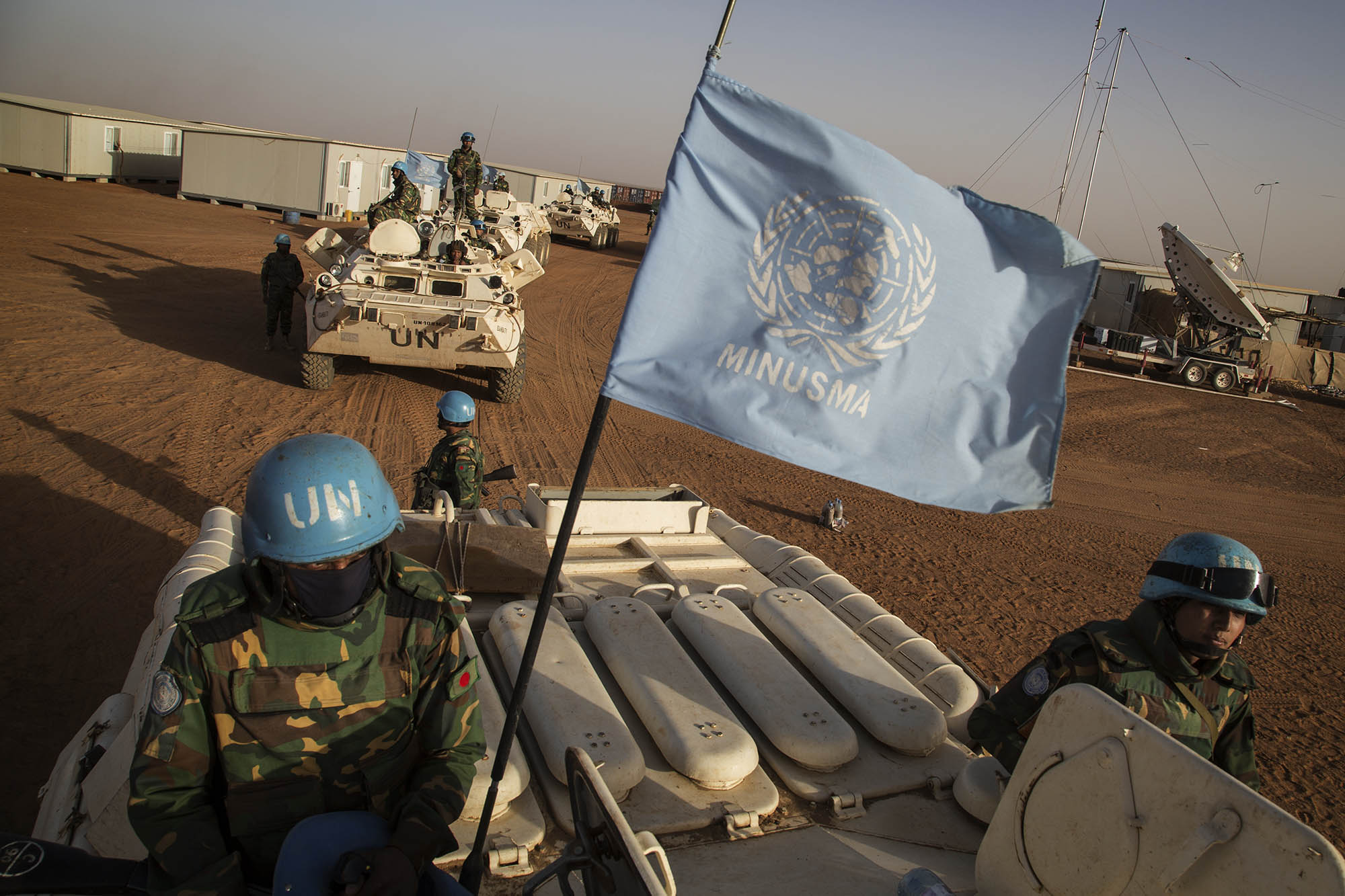In the foreground of the color photograph, a sandy field stretches out under a grayish sky. Dominating the scene is a convoy of UN vehicles, including what appears to be a golf cart-like vehicle at the front and several white tanks behind it. The vehicles are staffed by soldiers in camouflage uniforms, accented with blue UN helmets and face masks. One soldier stands behind the leading vehicle, vigilantly holding a gun. A light blue flag with a white emblem reading "M-I-N-U-S-M-A" flutters from the leading vehicle. The subsequent tanks also carry uniformed personnel. On the left side of the image, modern modular homes are visible, while on the right, a satellite dish and more mobile housing come into view. The overall terrain appears to be one of dirt and sand, and the light-colored modular buildings provide a stark contrast against the sky.